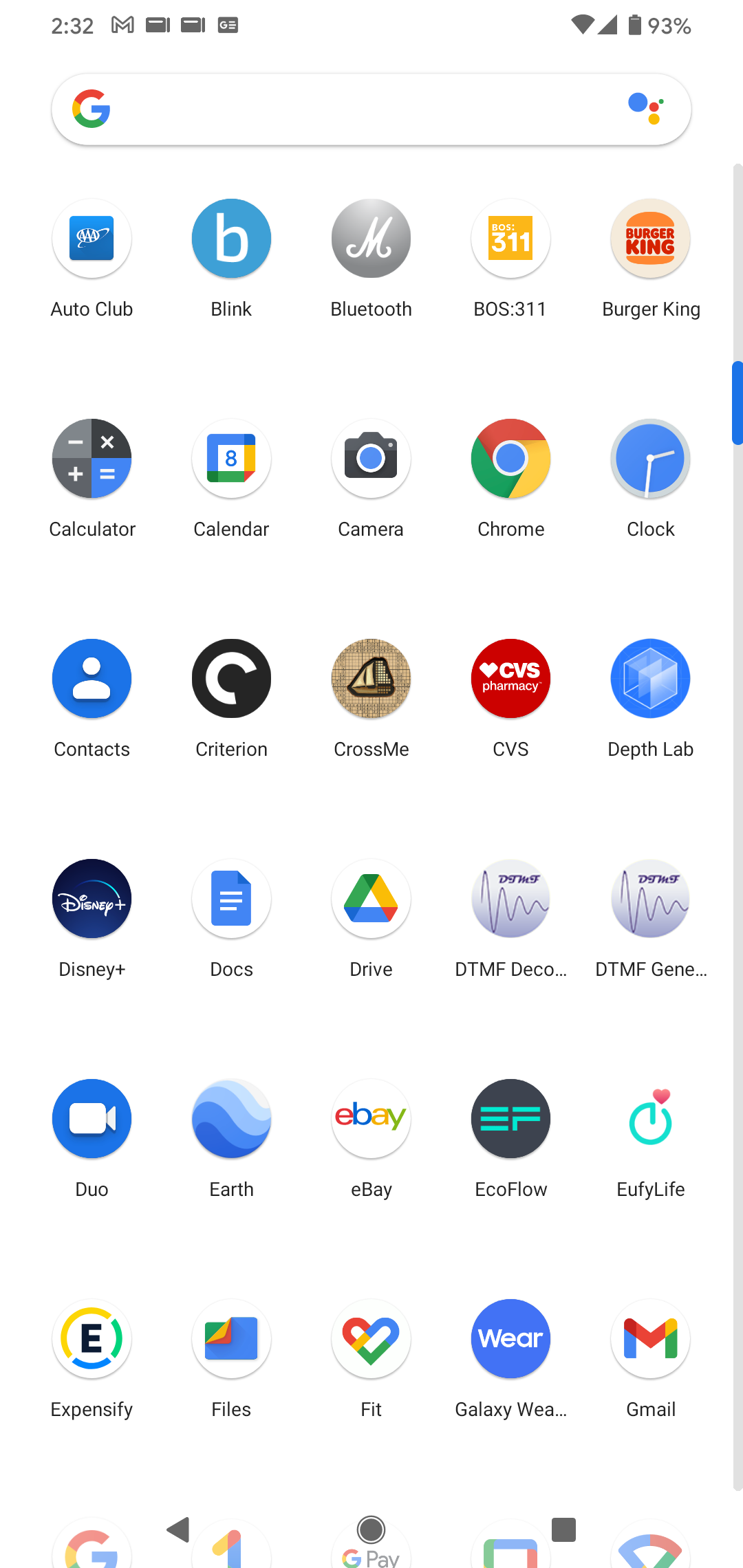This screenshot captures a cell phone's home screen with a variety of icons and features. At the top, the time reads 2:32, alongside a status bar displaying icons for Google Mail, Wi-Fi, and battery life at 93%. Beneath the Google search bar, a grid of app icons is visible.

From the top left, the icons are:
- AAA Auto Club
- Blink
- Bluetooth
- BOS 311
- Burger King
- Calculator
- Calendar
- Camera
- Chrome
- Clock
- Contacts
- Criterion
- CrossMe
- CVS
- Depth Lab
- Disney+
- Google Docs
- Google Drive
- DTMFDECO... followed by DTMFGene... (both cut off)
- Google Duo
- Google Earth
- eBay
- EcoFlow
- Eufy Life (capitalized as E-U-F-Y, L-I-F-E)
- Expensify
- Files
- Google Fit
- Galaxyware
- Gmail

At the bottom of the screen, there are several additional icons. These appear predominantly Google-based due to their color scheme, but the names are cut off and not visible in the provided screenshot. The arrangement and variety of apps give a detailed glimpse into the device's commonly used applications and functionalities.